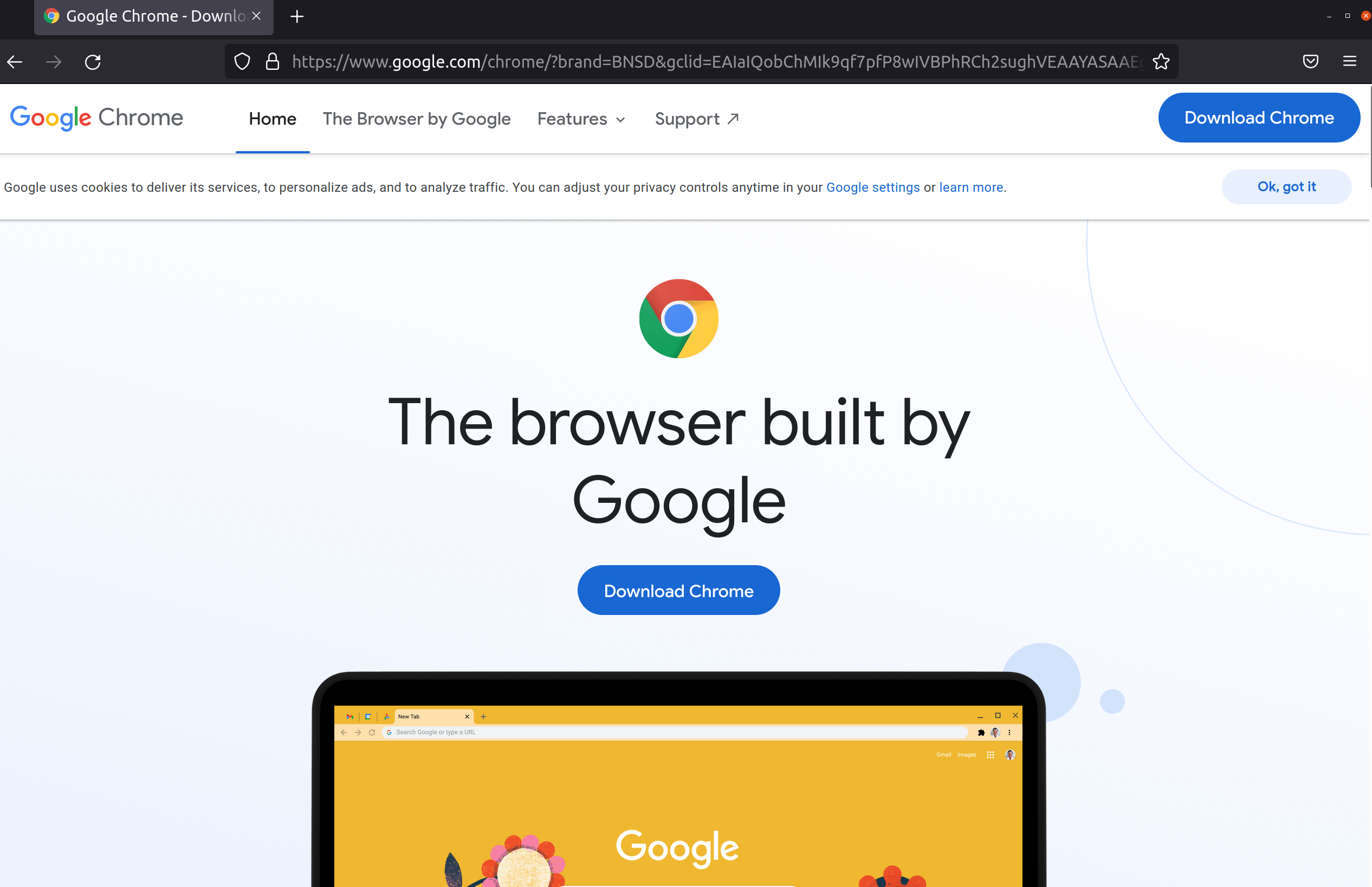The image displays a Google Chrome web browser open on a computer screen. At the top left corner, the label "Google Chrome" is prominently visible. To its right are multiple tabs titled "Home," "The Browser by Google," "Features," and "Support," with "Download Chrome" appearing at the far right. Below this navigation bar, a notification banner informs users about Google's use of cookies to deliver its services.

In the main content area of the browser, which has a white background with subtle circular designs on the right side, the Google Chrome logo—featuring red, green, yellow, and a blue center—stands out prominently at the top center. Directly beneath the logo, the text "The Browser Built by Google" is displayed, followed by a blue button with the white text "Download Chrome."

Below this call-to-action, the top half of a laptop screen is visible, showcasing another Google Chrome web browser window open within it.